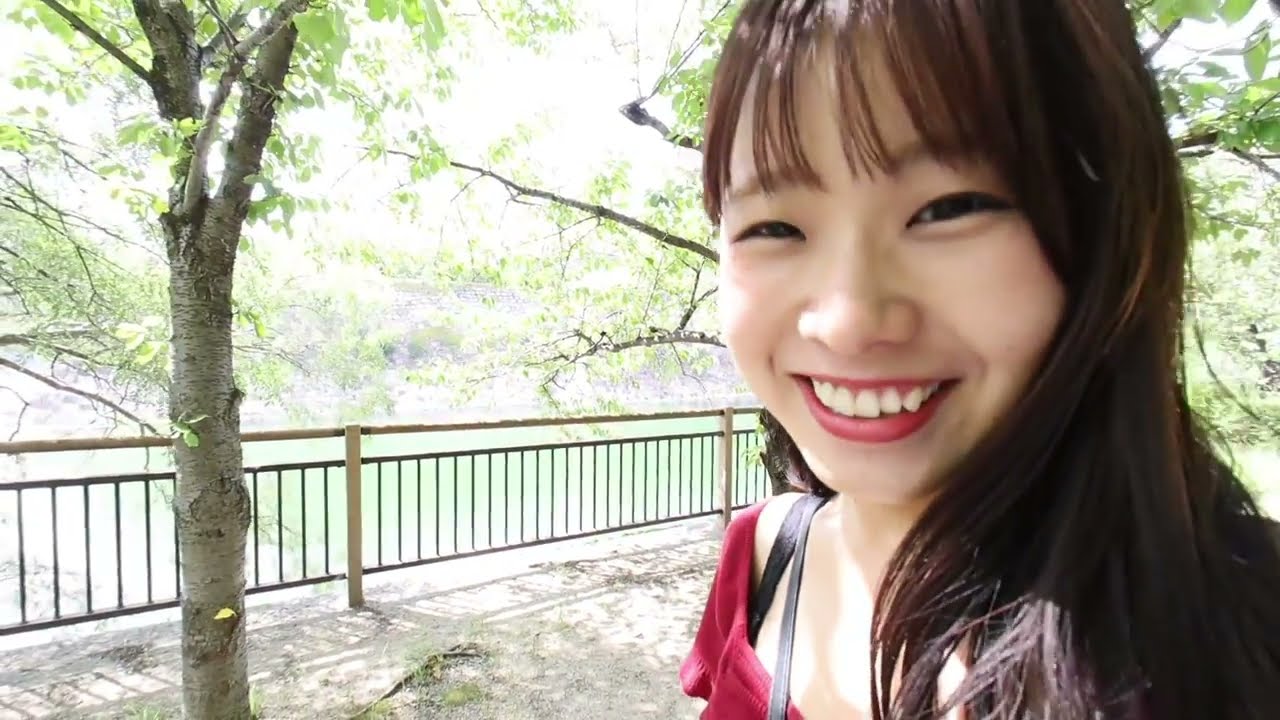In this vibrant outdoor summertime photo, a young Asian woman, likely in her early twenties, takes center stage with a radiant smile. Her dark, straight hair cascades down, accented by straight bangs framing her face. She's dressed in a red blouse, with visible black strap across her shoulder, indicative of a purse, and sports striking red lipstick. Her dark eyes sparkle with joy as she stands against a serene natural backdrop featuring a lush green tree to her left and a shiny steel guardrail. The ground immediately behind the guardrail is bare, marked by dirt, contrasting with the clear, greenish-blue river flowing beyond it. Further in the background, a softly sunlit, white-hued dirt hill adds a touch of tranquility to the hilly terrain, despite the obscured sky details.